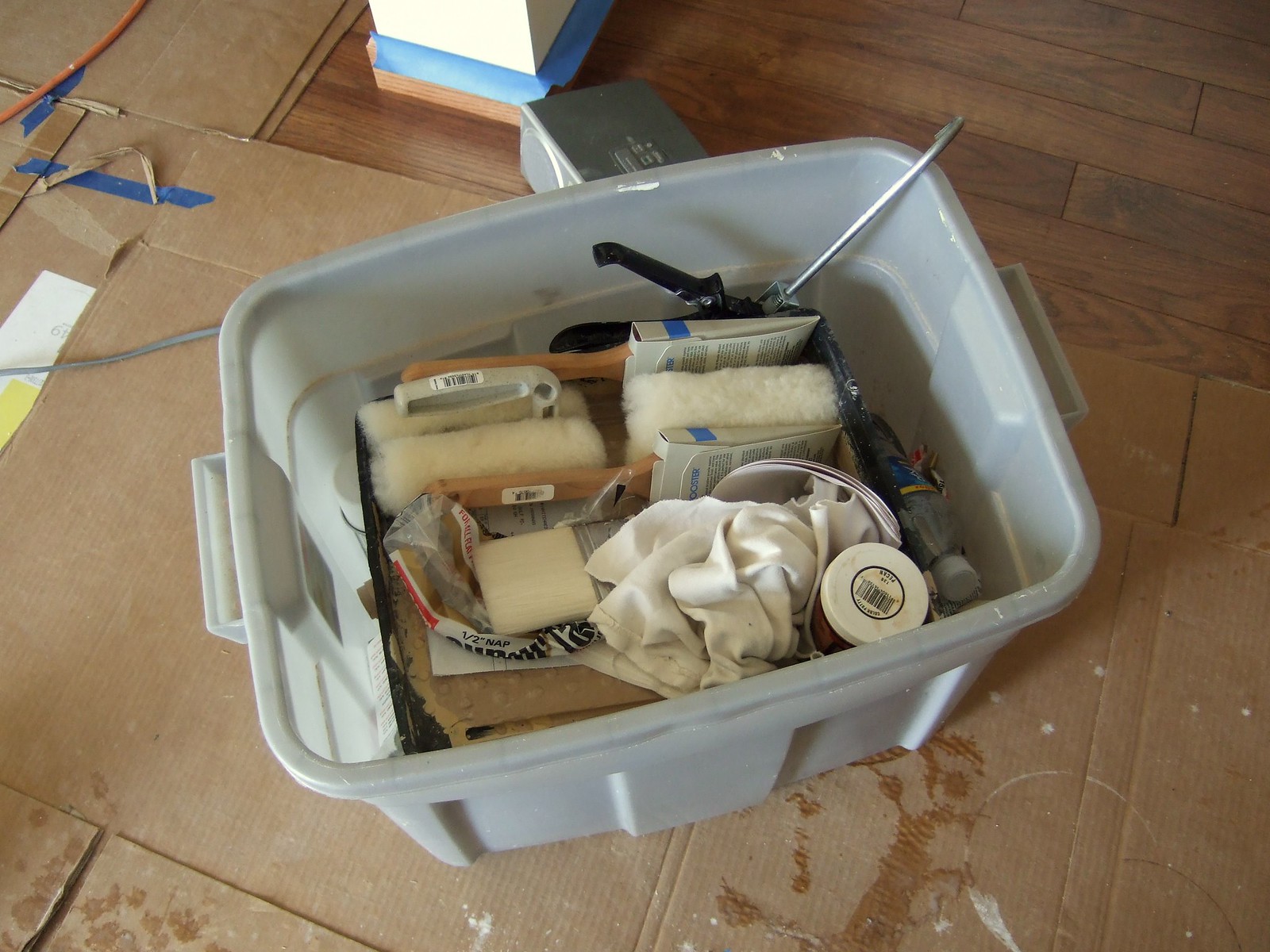The photograph showcases a scene of disarray on a brown wooden floor. A portion of a white wall is visible at the background. Scattered across the floor are flattened pieces of ripped-open cardboard boxes, some featuring blue markings. At the center of this scene is a gray plastic storage bin. Inside the bin, there is a clear bottle with a blue label and a white lid, a silver pointed object, and a brown paintbrush still encased in its original packaging. The bin also contains several white, puffy items, a white square item placed over a plastic bag which has a white label adorned with red and black writing. Adjacent to the bin, on the floor, lies a white towel and a jar with a white lid featuring a black circle with black writing on it.